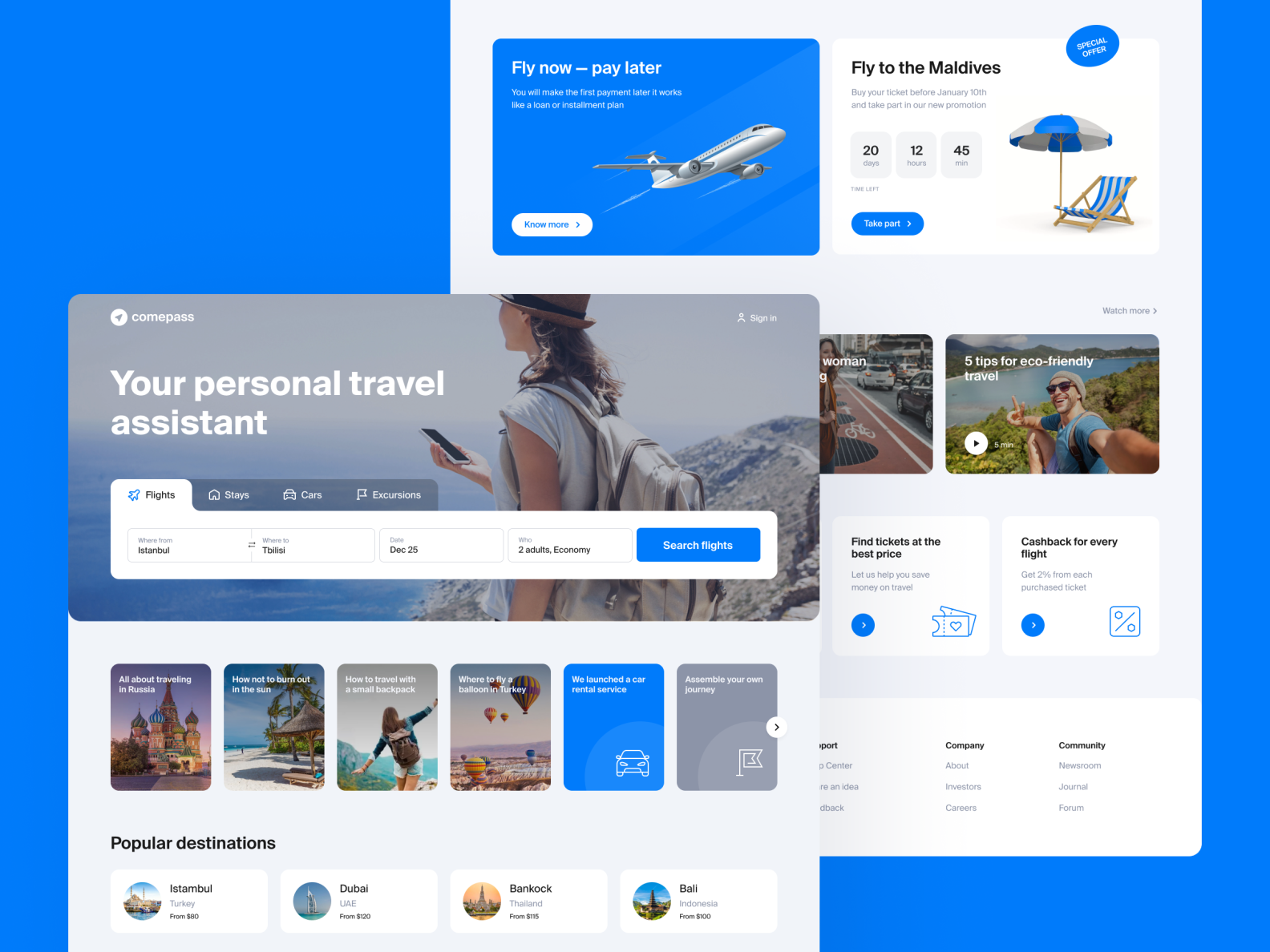The webpage appears to be a meticulously designed travel booking site, characterized by a predominantly blue and white color scheme and numerous overlays adding depth to the layout. At the top, a highlighted box reads "Fly Now, Pay Later," indicative of a flexible installment payment option for travelers. Adjacent to this, a vibrant section promotes "Fly to the Maldives," complete with figures like 20, 12, and 45 whose specific meaning isn’t immediately clear, alongside a visually appealing beach chair and umbrella, tempting viewers with the allure of the Maldives.

Centrally positioned on the page, a dedicated area titled "Your Personal Travel Agent" provides user-friendly navigation. It features selectable tabs for "Flights," "Stays," "Cars," and "Excursions," with "Flights" being the current focus, as indicated by its white background. This section includes interactive fields where users can specify their departure and destination locations, travel dates, and the number of travelers.

Below this, a series of thumbnail images captures diverse travel experiences: a majestic castle (possibly Disney-themed), a serene beach, a daring mountain climber, and colorful balloons being released. The bottom section of the page showcases "Popular Destinations," though only Dubai is decipherable among the listings due to overlay obstructions. Additionally, a video titled "Five Tips for Eco-Friendly Travel" hints at sustainable travel advice.